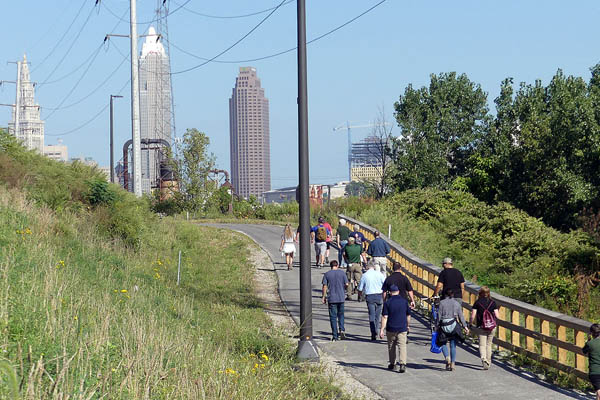This color photograph captures a bustling scene of pedestrians walking away from the camera on an asphalt pathway that curves to the left and disappears into the distance. The pathway begins at the lower right corner of the image, flanked on the left by a grassy hillside adorned with yellow wildflowers and shrubs. A wooden railing, accompanied by a black metal post, runs alongside the right of the path, adding structure to the scene. Tall power lines stretch across the skyline, anchored by large posts visible just past the hill. Among the diverse crowd are men and women in casual attire, some carrying backpacks and bags. The bright, clear blue sky serves as a backdrop for a cluster of office towers, including three prominent buildings on the left and another under construction on the right, complete with a crane. To the far right, verdant green trees complete this vivid portrayal of city life on a sunny day.